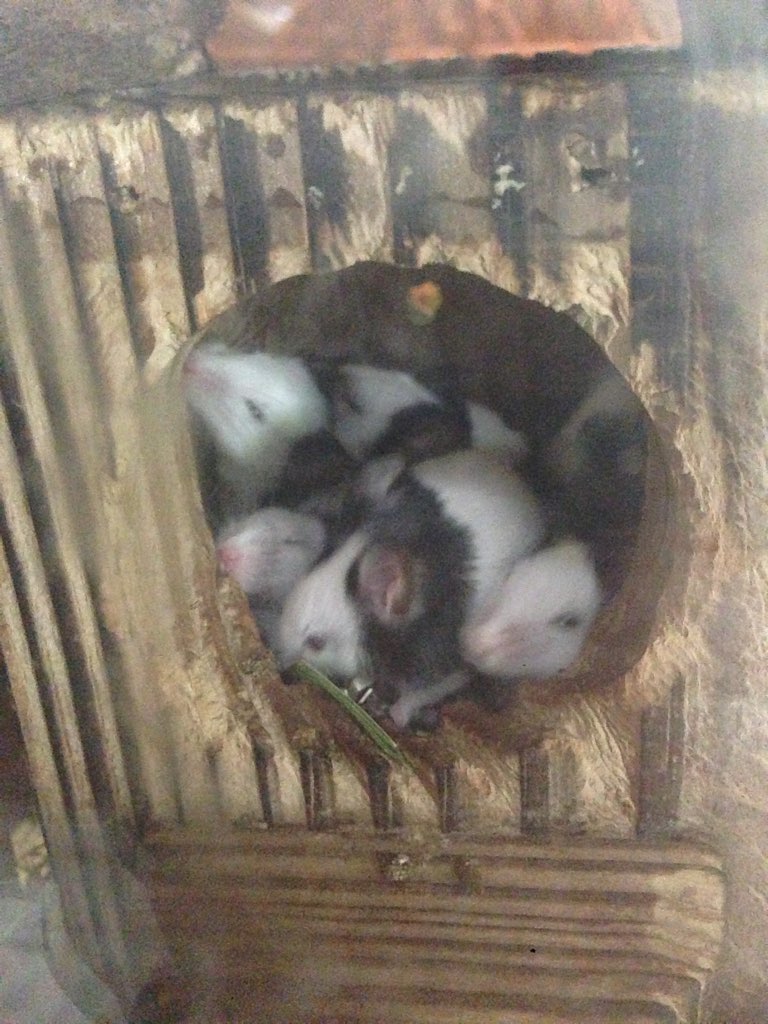The image is a vertical rectangle-shaped photograph capturing small rodent-like animals nestled inside a rough, irregularly carved hole within a wooden structure. The wood, resembling a tree trunk or perhaps wooden furniture with a shelf-like bottom, features a mix of horizontal and vertical black lines. Adding to the intricate details, the top of the frame shows a red, brick-like element, possibly part of the structure. Patches of grass are visible within the hole, further grounding their natural nest. Approximately five to six black-and-white rodents with pink noses, pink ears, white whiskers, and black eyes huddle together. One rodent peeks through another hole at the back, revealing a little yellow flower sticker. The photograph, slightly blurred, portrays a cozy, nature-integrated dwelling for these small creatures.